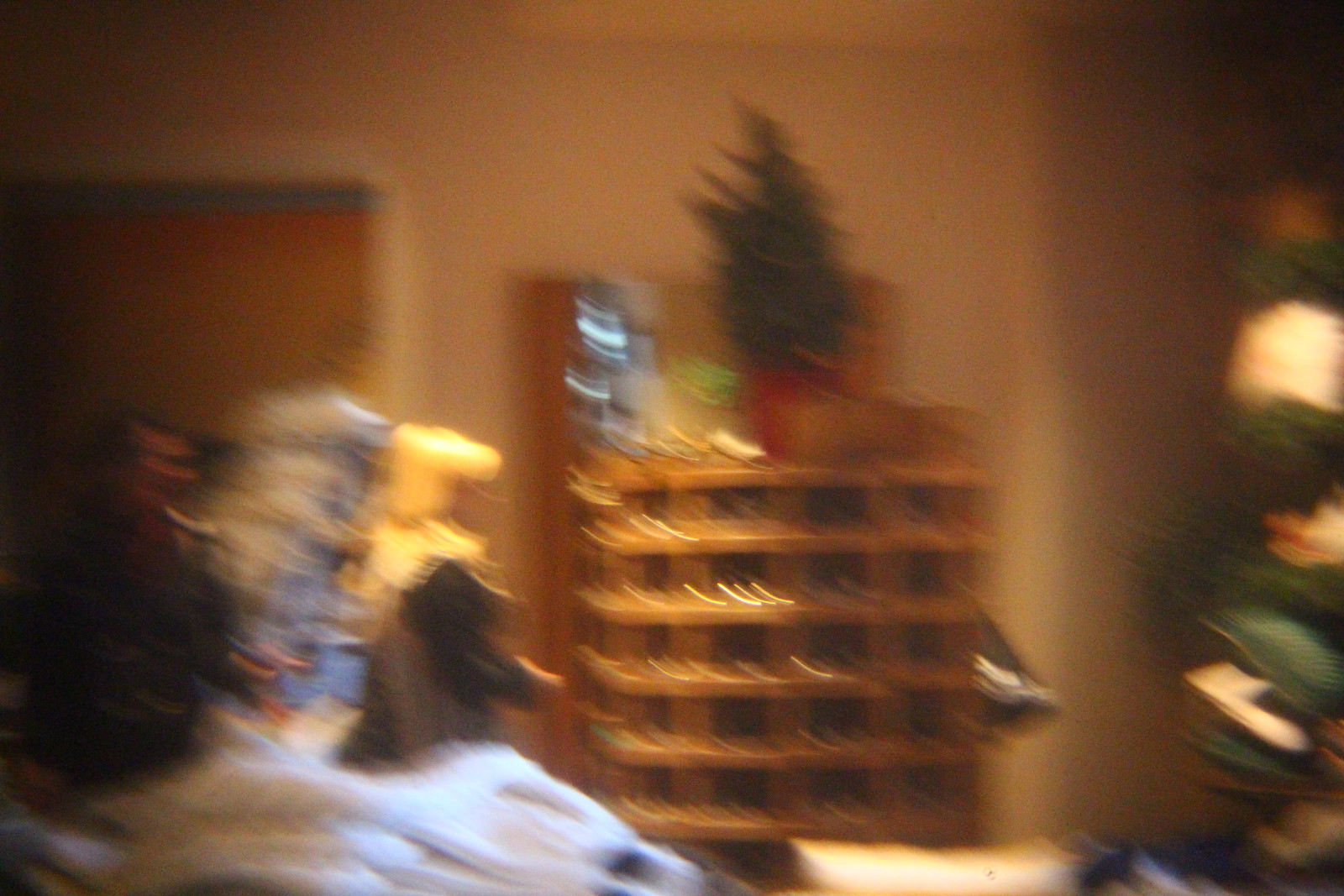This extremely blurry photograph appears to be taken indoors during the holiday season. Central to the image, there is a small Christmas tree, possibly an artificial one about 2 feet high, placed on top of what looks like a wooden wine rack with square slots, suggesting it may hold bottles or other items. The tree is in a red pot and stands among various indiscernible objects on the rack. To the left, there's what appears to be a door with possibly a bed or a couch in front of it, covered by a light blue blanket. The right side of the image is also blurry, but there might be another Christmas tree extending up. The photograph is notably unclear, making many details difficult to discern.